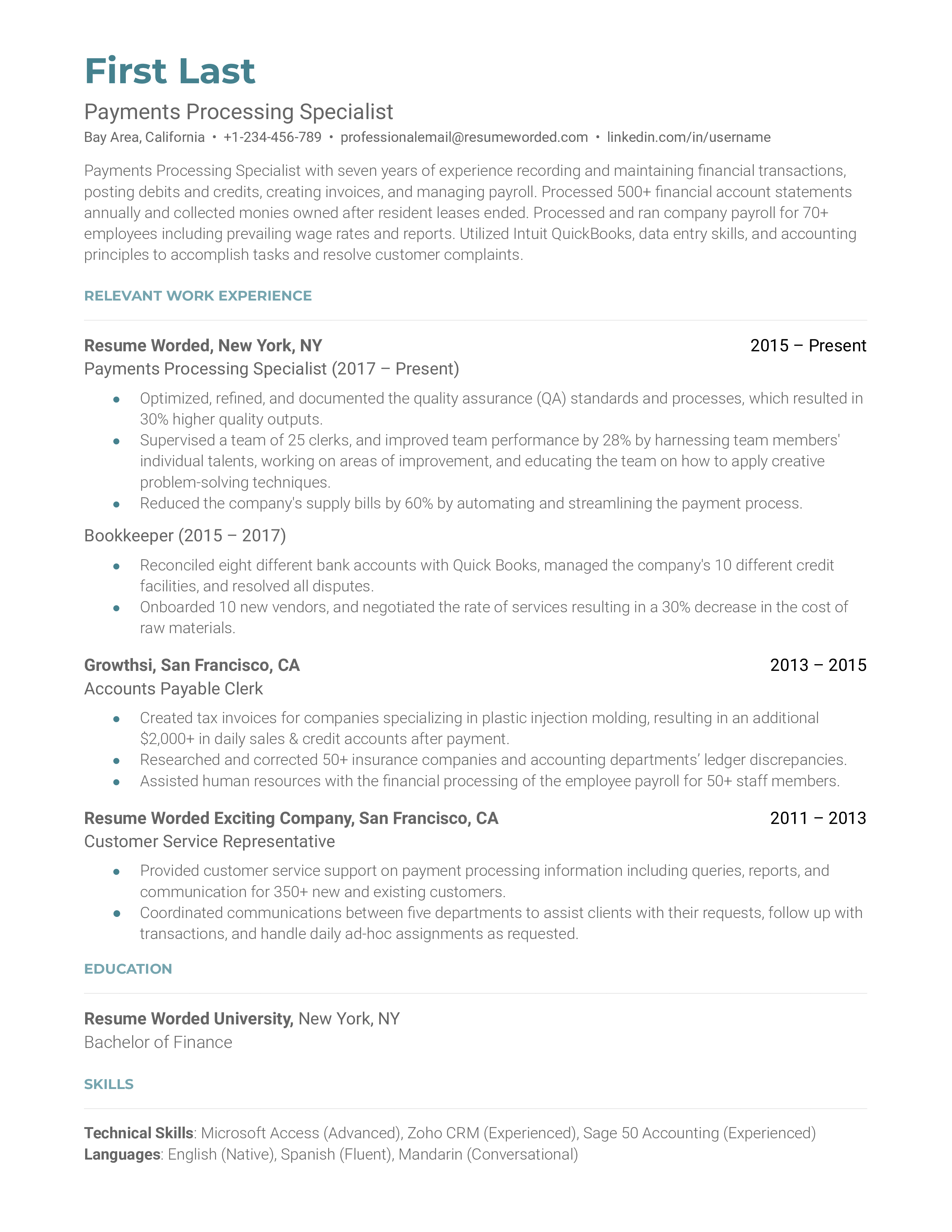The image depicts a professional and meticulously designed resume template tailored for a Payments Processing Specialist based in the Bay Area, California. At the top left corner, the name "First Last" is prominently displayed in medium blue letters. Below the name in black letters is the job title, Payments Processing Specialist, followed by the location, Bay Area, California, and contact information including a phone number, professional email, and LinkedIn profile.

The resume is structured into distinct sections, each highlighted with blue category titles and black font text, showing a clear and professional layout. It features a detailed summary emphasizing the candidate's 7 years of experience in recording and maintaining financial transactions, posting debits and credits, creating invoices, managing payroll, processing over 500 financial account statements annually, and other key responsibilities. Specific accomplishments include collecting owed monies after lease terminations and managing payroll for 70+ employees, including prevailing wage rates and reports, all executed using Intuit QuickBooks and robust accounting principles.

Further down, the template allocates space for listing relevant work experiences, evidenced by bullet points that summarize high points of previous positions, details of employment organized on the right side. An education section follows, intended for academic history and relevant coursework, and finally, a skills section at the bottom allows for the inclusion of technical skills, languages, and other pertinent abilities. The overall appearance of the resume is very professional with neatly organized sections and a clean, easily readable font.